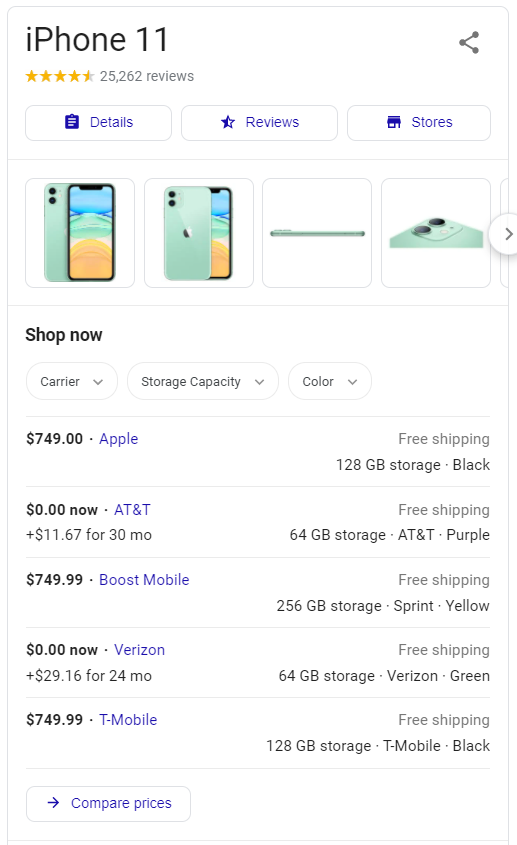The image is a screen capture from a mobile device with a white background. At the upper left corner, "iPhone 11" is written, accompanied by four and a half yellow stars and the text "25,262 reviews" beside the stars. Beneath this information, three horizontally aligned rectangular buttons are displayed, labeled "Details," "Reviews," and "Stalls" in blue text.

Below these buttons are four images of a pastel green-colored cell phone. Underneath the images, the phrase "Shop Now" appears in black text. A row of three drop-down buttons follows this, labeled "Carrier," "Storage Capacity," and "Color" from left to right. At the bottom are various listed prices for the product.